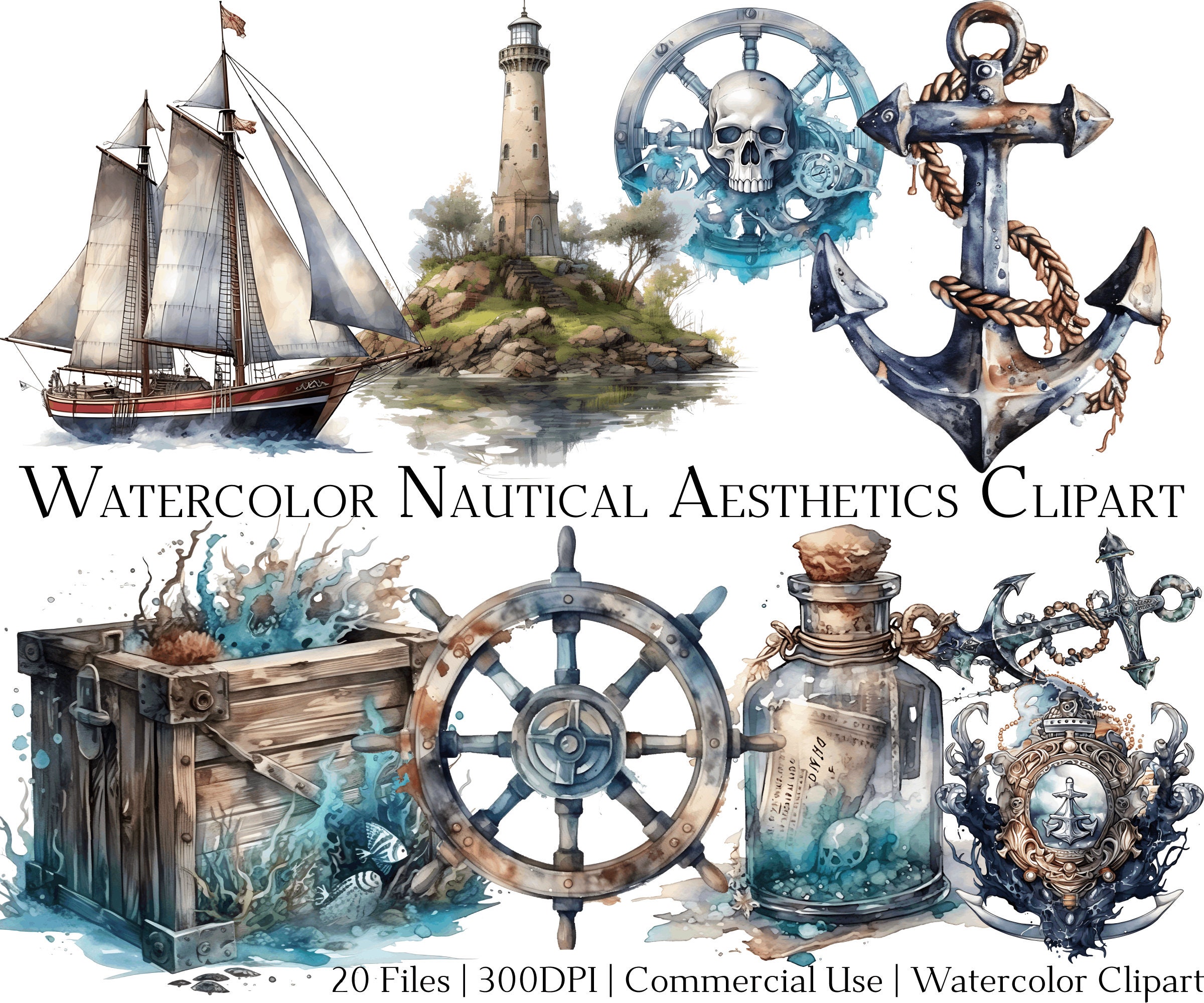The image depicts a poster featuring the text "Watercolor Nautical Aesthetic Clipart," promoting 20 files available at 300 dpi for commercial use. The poster is set against a white background, and its core visuals are in tones of sea green, browns, and some greens. At the top, there are four primary images: a tall ship with big white sails and a small flag at the top, a lighthouse on a hill, a ship's wheel with a skeleton in the center, and a silver anchor partially rusted and wrapped in rope. Below the text, additional images include an old trunk or treasure chest with sea plants and seashells growing out, a captain's wheel, a message in a bottle, and a silver crown with an anchor atop. The nautical-themed clip art encompasses elements like sailboats, a ship wheel, a message in a bottle, and an anchor, all rendered in a watercolor aesthetic.